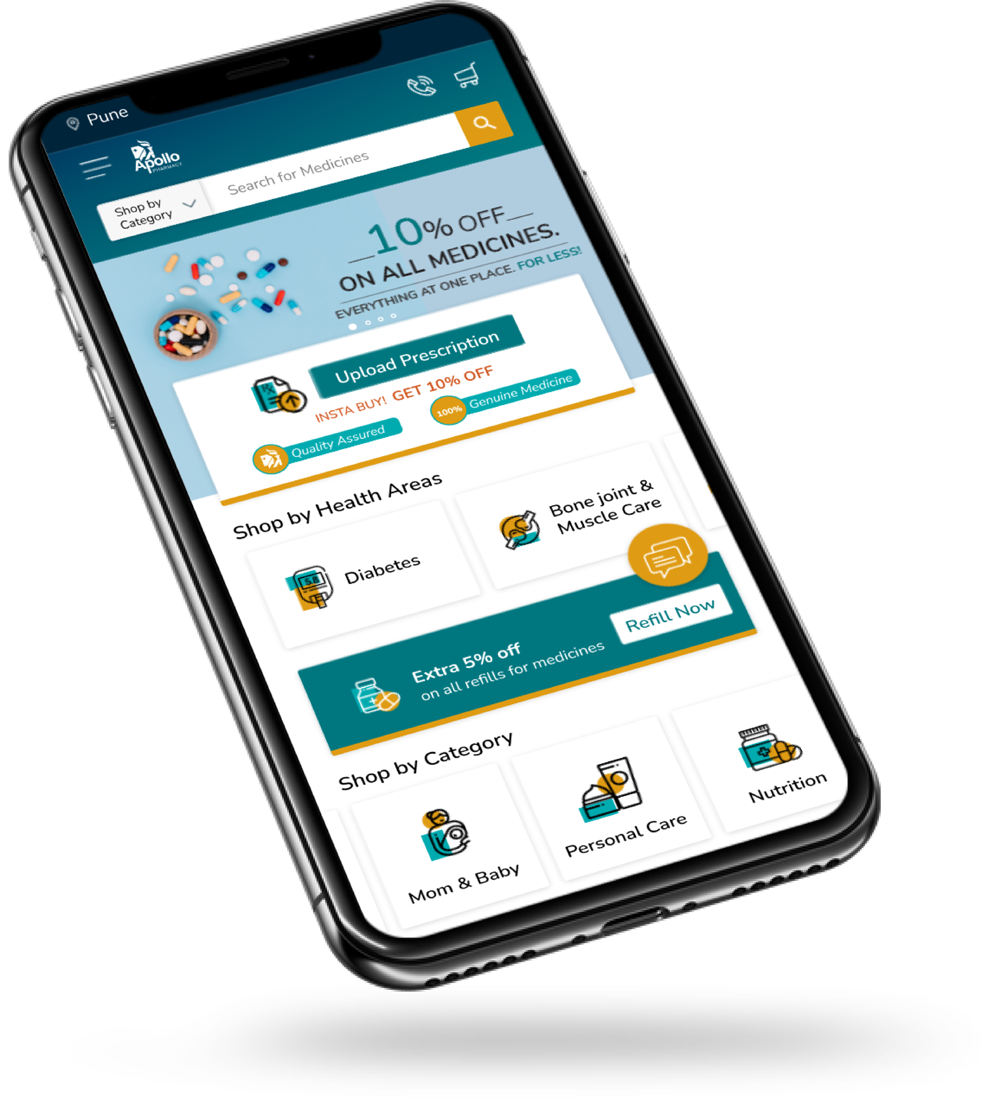In this image, a smartphone screen displays a prescription medication website from Apollo. The top of the screen features a distinct green bar with 'Apollo' written on it. Adjacent to this, the top left section remains white, containing three horizontal lines that represent the menu button. The top right holds icons for a phone and a shopping cart. Directly underneath is a white search bar that reads 'shop by category' on the left, accompanied by a drop-down arrow, and an orange search button on the right. Below this, a light blue banner showcases scattered pills and prominently offers a "10% off on all medicines" deal, with the number 10 in green and the rest of the text in black. Following this, a large white rectangle holds center stage, featuring a green button labeled 'Upload Prescription' in its middle. Beneath this button, an orange text advertises a buy one get one 10% off promotion. At the very bottom of the screen, the phrases 'quality assured' and 'genuine medicine' are printed in orange, separated by an orange line.